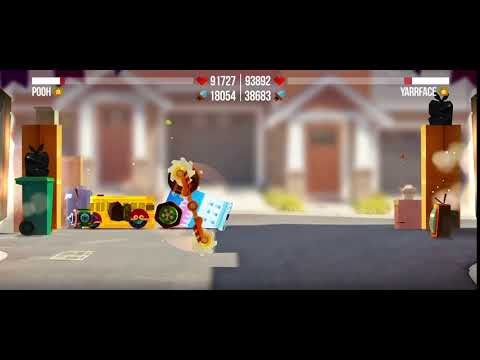This image is a low-resolution screenshot of a video game featuring a chaotic urban scene. The screen is framed with thick black borders at the top and bottom. At the top of the screen, the word "POOH" is displayed alongside a series of numbers: 91727, 93892, 18054, and 38683. In the upper right corner, the name "YARFACE" is visible.

The background of the image is blurred, depicting a series of houses or garages. A noticeable detail in the center foreground is a blue shape with wheels, likely some kind of vehicle, possibly battling another vehicle featuring saw blades, rockets, and other makeshift, menacing contraptions. This combat theme is reinforced by the presence of two white horizontal bars at the top, resembling health bars seen in fighting games, as well as numbers accompanied by red hearts and swords.

On the right-hand side, there's a green trash can topped with a black trash bag. Two brown columns are positioned in the background, and clutter is scattered around them, making the scene appear disorderly. This clutter includes items that resemble lottery tickets and buttons. Toward the center, there's a large wooden stick-like object with a circular saw blade affixed to it. Another detail on the right side is an old tube CRT television with black antennas sitting on the floor. The overall scene is set against a floor that intermixes light and dark gray tones, further emphasizing the gritty, chaotic atmosphere of the game.